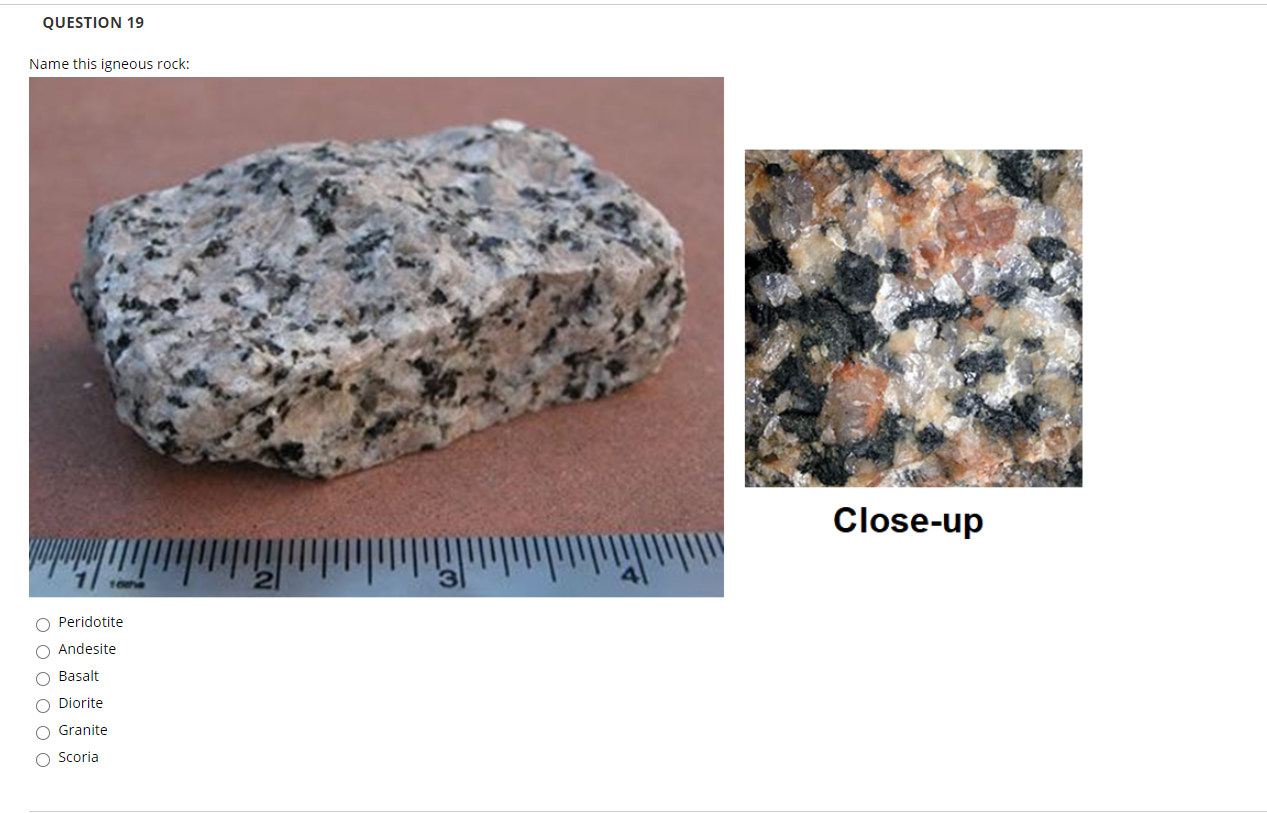This image depicts a quiz question labeled "Question 19" in small black lettering at the top left. Below this, the prompt "Name this igneous rock" is given. Dominating the center is a large square photograph of a tan rock speckled with black, white, and some hints of pinkish-gray flecks. In the foreground of the photo lies a metal ruler marked from 1 to 4 inches, suggesting the rock is around 4 inches in length. The rock is set against a red background. Beneath this main image are multiple-choice bubbles with the options: peridot, andesite, basalt, diorite, granite, and scoria. To the right of the main image is a smaller square labeled "Close up" in large letters, featuring a detailed view of the rock's speckled composition.